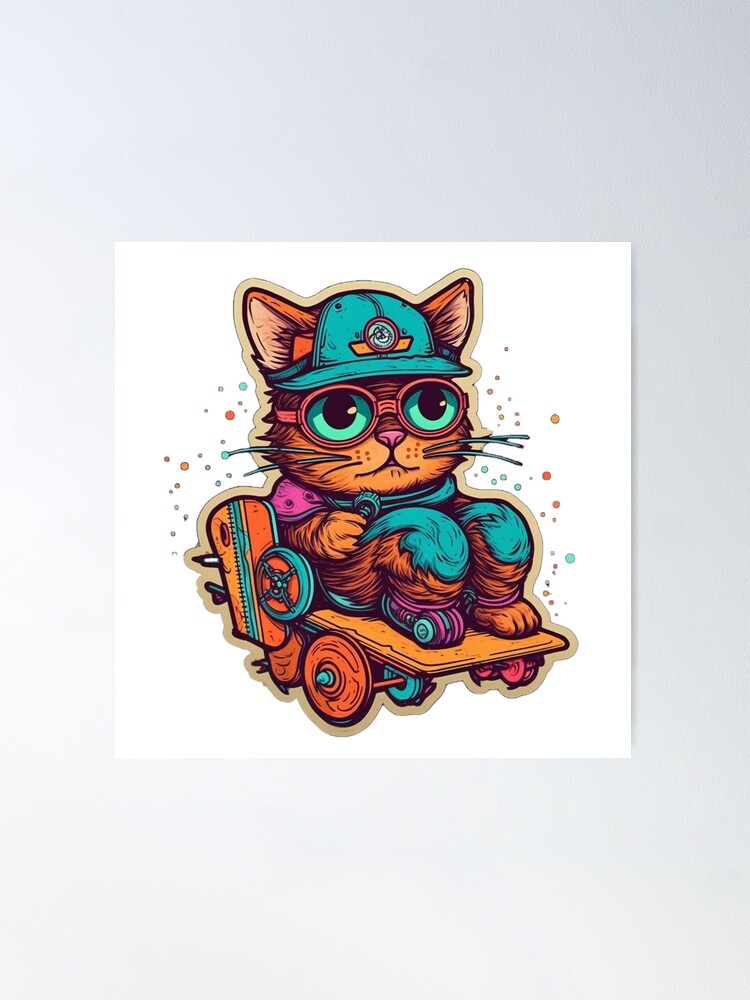This illustration presents a playful and whimsical orange-brown cartoon cat with prominent blue eyes set behind large goggles. The cat sports a turquoise baseball cap with ears peeking out, matching turquoise knee pads, and possibly even something on its paws. Seated as if mimicking a human, the cat perches on a wide board resembling a hybrid between a skateboard and scooter. This board, primarily brown with blue accents, features a variety of wheels, including an axle with two visible front wheels, while the rear wheels remain obscure. The entire scene is set against a white background, dotted with small bubbles, enhancing the playful and lively atmosphere of this detailed artwork.